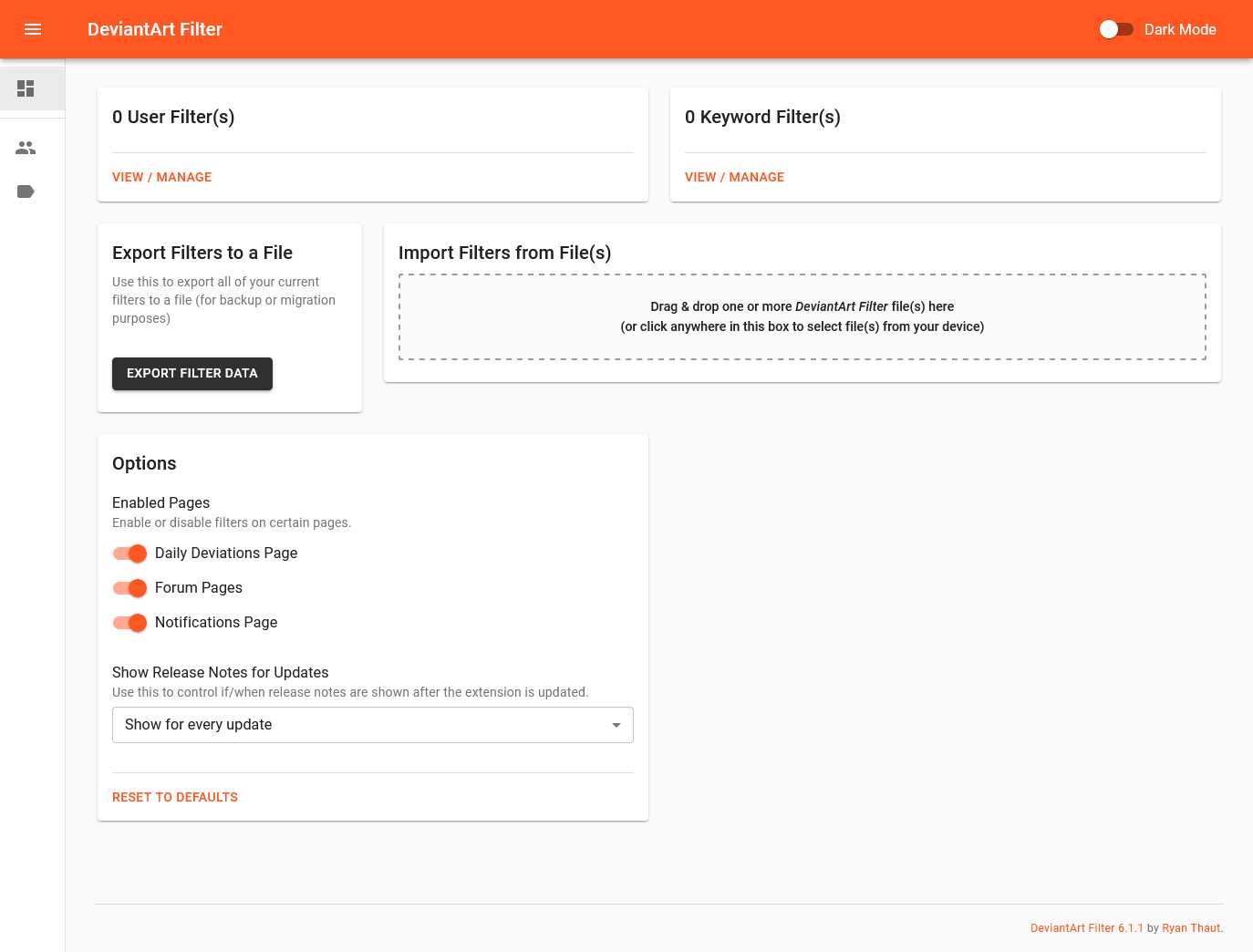**Detailed Descriptive Caption:**

The image depicts a web application interface with a Material Design theme, prominently featuring an orange header, suggesting that orange is the primary color scheme. The web application is titled "DeviantArt Filter."

On the left sidebar, three icons are visible, with the first, a gallery or grid icon, currently selected. The other two icons resemble a user icon and a battery icon with ambiguous details. 

The main content area displays several panels and cards: 

1. A card reading "Zero User Filters" with an option "View / Manage" at the bottom. 
2. Another card labeled "Zero Keyword Filters" also featuring a "View / Manage" option.
3. A card titled "Export Filters to a File" explaining its functionality: "Use this to export all your current filters to a source file for backup or migration purposes."
4. Another card on the right, named "Import Filters from Files," instructing users to "Drag and drop one or more DeviantArt filter files here to begin with a new device."
5. The final card at the bottom, titled "Options," lists several toggles: "Enable daily aviation pages," "Enable form pages," "Enable notification pages," and includes an option to "Show release notes for every update." There are also "Reset" and "Default" buttons at the bottom for restoring settings.

The footer of the interface shows the application version "DeviantArt Filter 6.1.1" and credits the developer "Ryan.CHAUT."